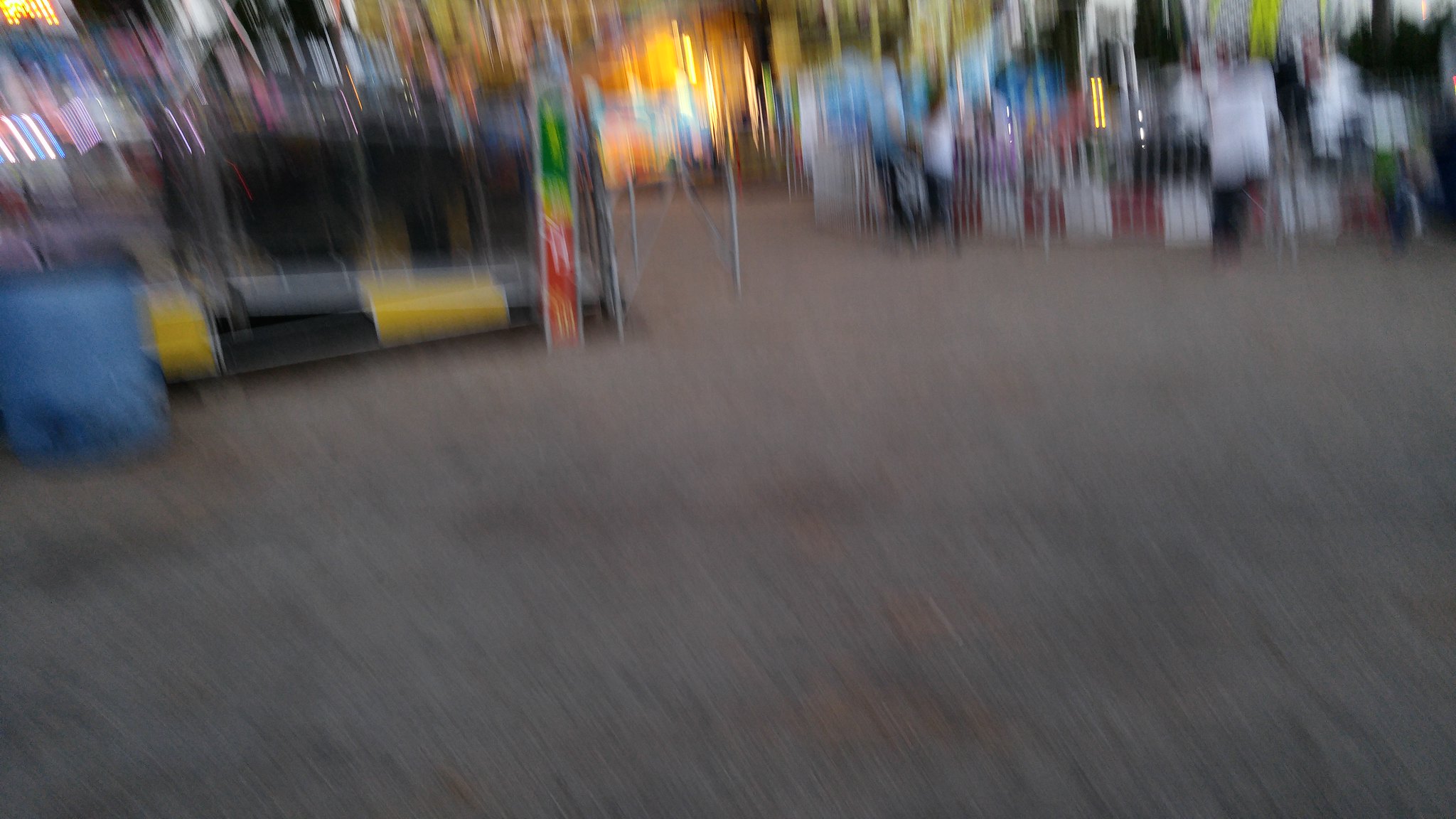This image captures an exceptionally blurry outdoor scene, resembling a fairground or carnival. The photograph is taken in a landscape format and is disorientingly out of focus, featuring vertical lines of blur that dominate the composition. The foreground, which occupies about two-thirds of the image, displays a mixture of light brown and gray ground—likely dirt, sand, or cement, interspersed with darker brown patches. In the background, illuminated areas splash various colors against the haze: primarily yellow, blue, and orange lights that suggest evening or early morning lighting. Distinct amidst the blur, a yellow and black striped bumper, possibly part of a ride, stands out alongside a tarped section. A notable detail includes a small sign or part of a structure that displays red at the bottom and green at the top. On both sides of the image are indistinct structures, possibly game stands or amusement rides, contributing to the fairground atmosphere. Scattered within the blur are figures of people, distinguishable by their white shirts and dark pants, enhancing this sense of a bustling, albeit unclear, scene.